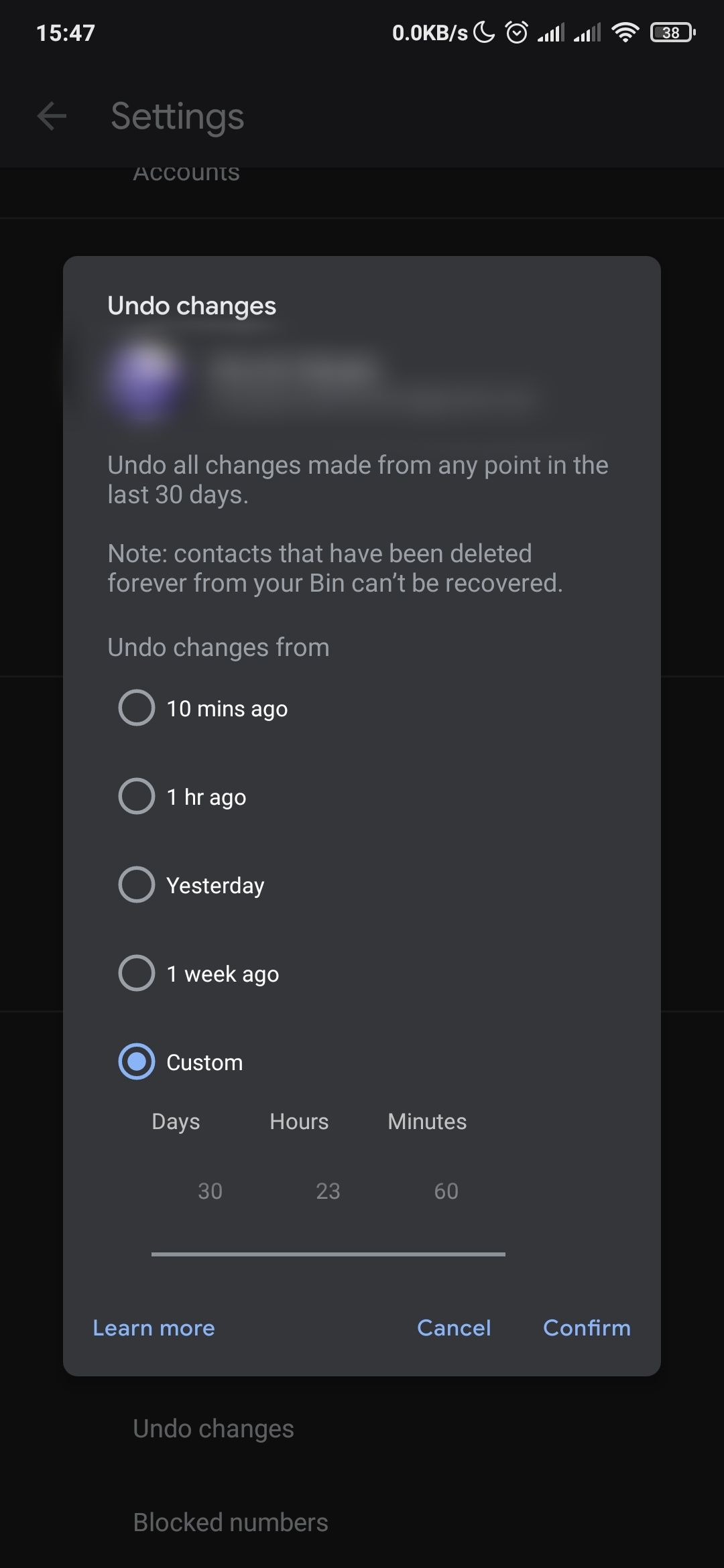A screenshot from a smartphone displays the device's settings interface against a dark black background. A semi-transparent grey pop-up window occupies the central focus, featuring light grey text. The pop-up is titled "Undo changes" and includes a partially blurred message that reads, "Undo all changes made from any point in the last 30 days. Note: Contacts that have been deleted forever from your bin can't be recovered." Beneath this message, there are five selectable options with circular buttons next to each: "10 minutes ago," "1 hour ago," "yesterday," "1 week ago," and "custom." The "custom" option is selected, indicated by a blue highlighted circle with a dot in the center. Below this section, the text reads "30 days, 23 hours, and 60 minutes."

Further options at the bottom of the pop-up include "Learn more," "Cancel," and "Confirm." The upper-left portion of the screen shows the word "Settings" with a left-pointing arrow to navigate back. At the bottom beneath the pop-up, partially visible text reads "Undo changes" and "Block numbers."

In the status bar at the top of the screen, the time is displayed as 15:47. The top-right corner shows the Wi-Fi icon, battery level at 38%, and an alarm clock symbol.